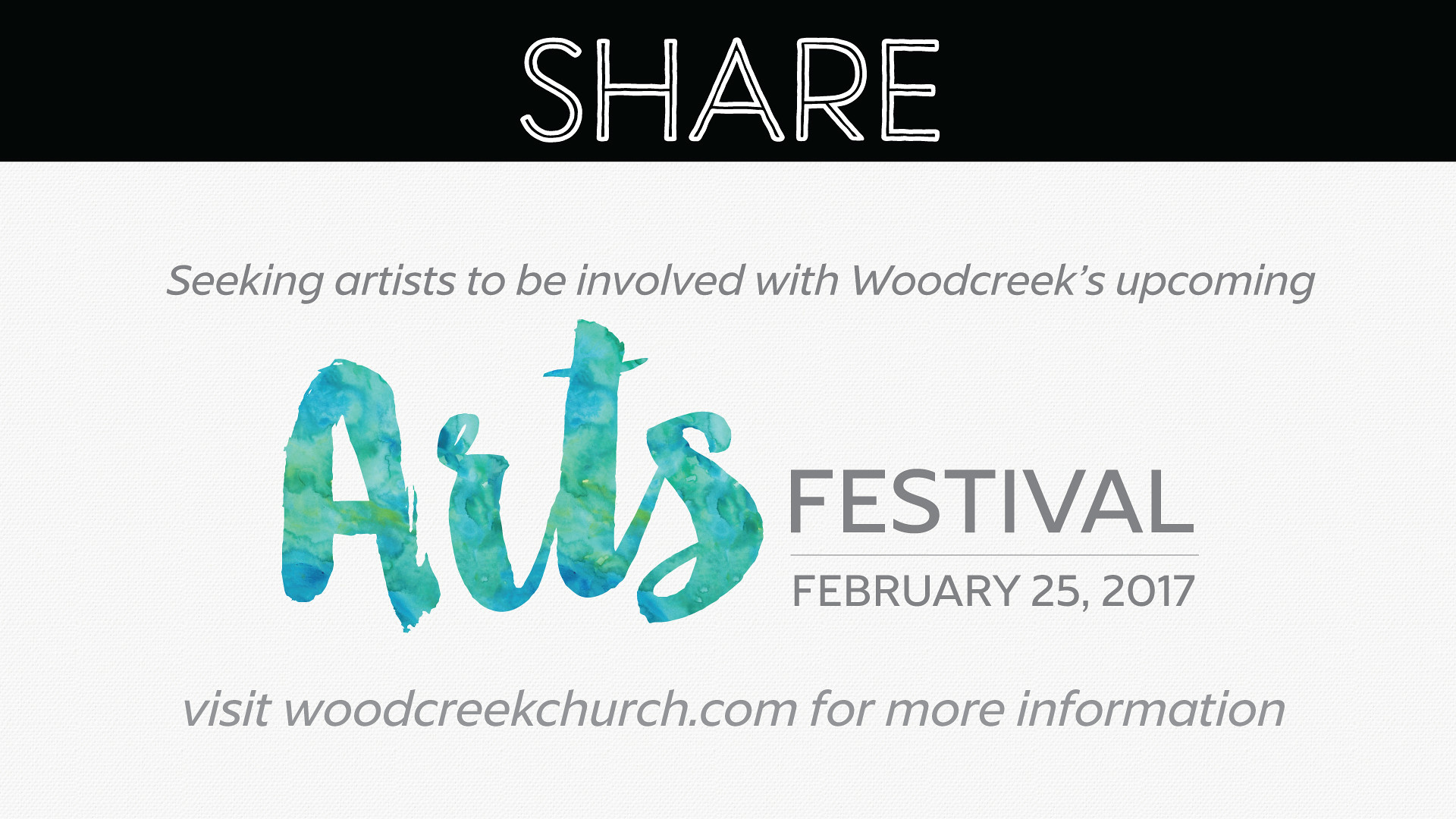This image is a landscape-oriented flyer designed to promote an arts festival. At the top, there is a black bar occupying roughly 15% of the height, featuring the word "SHARE" in prominent double white font. The remainder of the flyer’s background is white. Below the black banner, gray text reads: "SEEKING ARTISTS TO BE INVOLVED WITH WOODCREEK'S UPCOMING." Centrally, the word "ARTS" stands out in a vibrant, bluish-greenish paint-style font with a multi-swirling color effect within its thick, see-through letters. Beneath "ARTS," the word "FESTIVAL" is displayed in dark gray capital letters, followed by "February 25, 2017." At the very bottom, the flyer directs viewers to visit "woodcreekchurch.com for more information." This visually appealing announcement seems intended for sharing on social media to garner attention and participation in Woodcreek's Arts Festival.